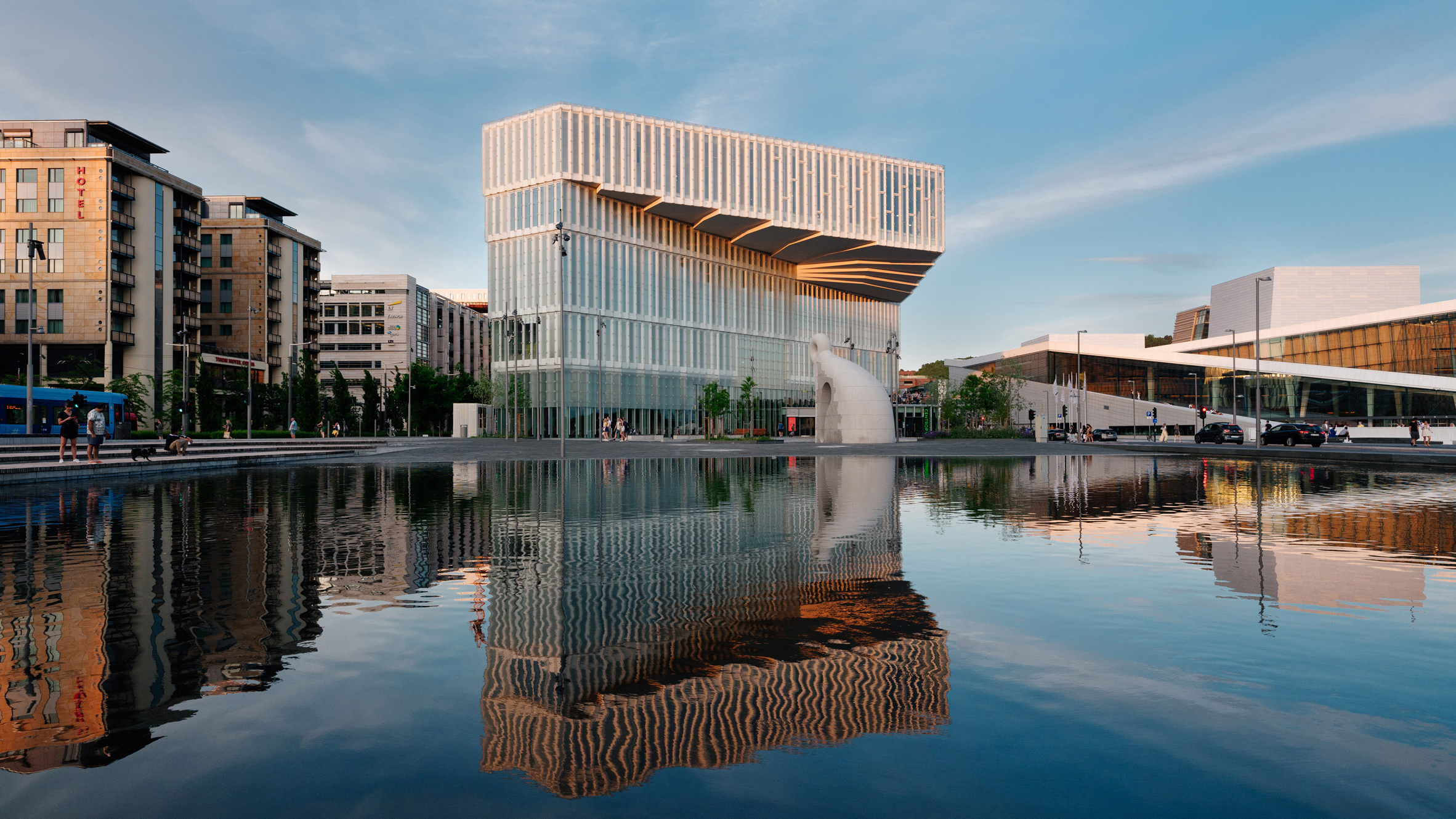The photograph captures a vibrant urban scene viewed from across a calm, reflective body of water, which could be a large pond or a flooded area. The water is so smooth it creates a near-perfect vertical reflection of the skyline. In the foreground, there are several people, some walking dogs, others taking photographs. Notable in the background is a dense array of buildings with distinct architectural features.

On the left side, there are modern brownish-white high-rise buildings, including one labeled "Hotel" in red text, another with balconies, and a bright blue bus passing by. Further back is a grey building resembling a parking garage, and an unusual white metal and glass building whose top floor slightly overhangs with a unique pattern, reminiscent of an open hand of cards. This building is centered and has somewhat of a vent-like design, topped by an odd-shaped white structure – possibly an art installation.

To the right of this striking building, there's a slightly angled white edifice with brown windows beside a road where multiple cars are parked. A walkway lines the water, where more pedestrians are seen strolling. The sky is a lovely blue with streaks of white and grey clouds, indicating daytime, probably late in the afternoon. The whole scene is bathed in bright natural light, adding clarity to every detail, from the skyscrapers and crosswalks to the trees lining the streets.